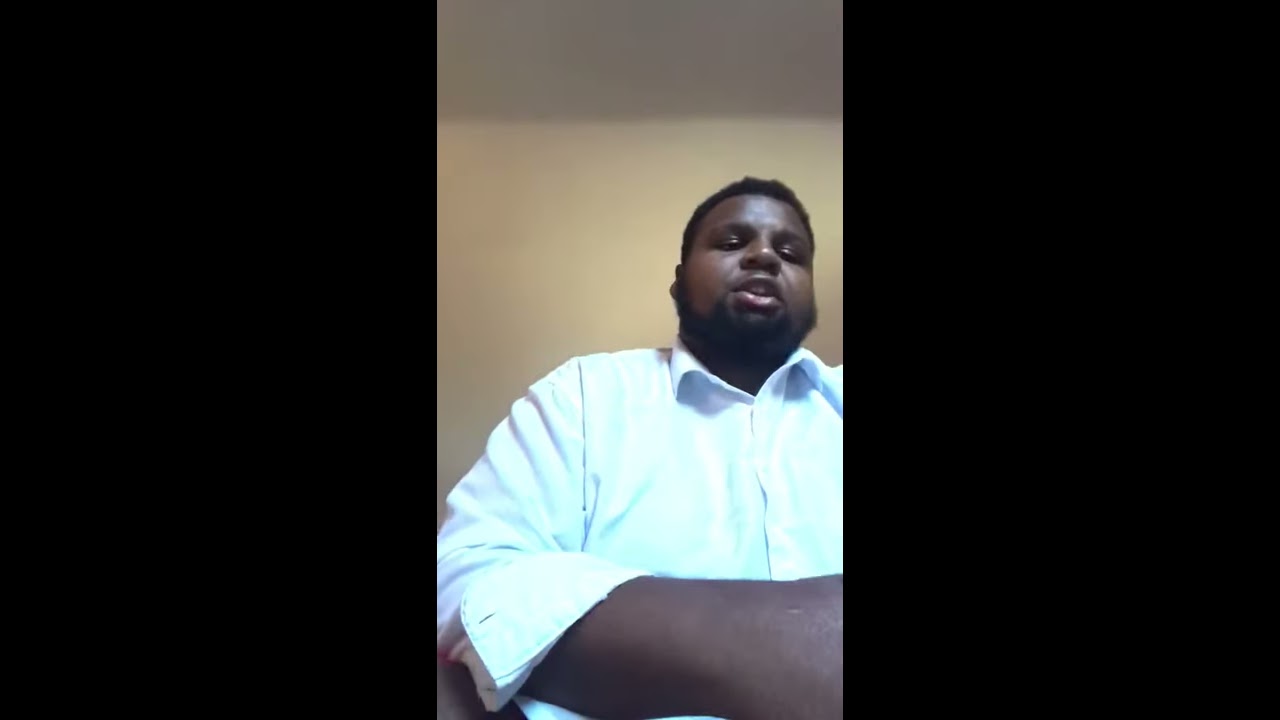This image captures a close-up of an African American man with short, dark hair and a short beard or goatee, possibly with a thin mustache. His facial expression suggests he is either talking or looking downward. He is dressed in a white or light blue collared shirt, buttoned to the top with the collar slightly open. The shirt appears somewhat cuffed back, revealing part of his right arm and hand, which is the closest element to the viewer, foreshortened due to the camera angle. The photograph, likely taken with a cell phone, features substantial black rectangular spaces on both the left and right sides, framing the central image of the man. The background is a cream or darker tan wall, relatively plain except for a subtle shadow at the top.